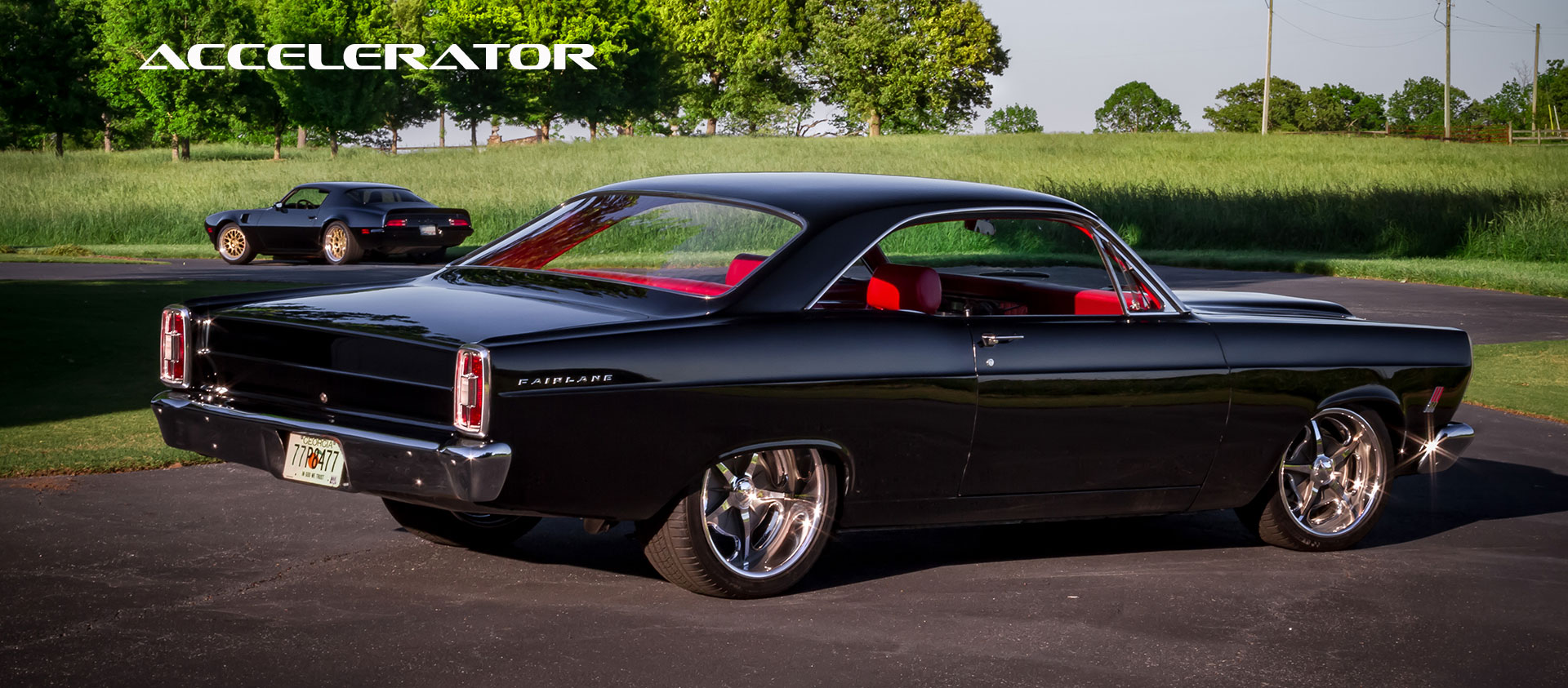This professional photograph features a meticulously maintained classic black Ford Fairlane with a sleek and shiny exterior. The view captures the vehicle from the right-hand side, revealing its angular build and high-quality, extra wide wheels with shiny chrome hubcaps partially covered by the frame. The car boasts a lustrous red leather interior visible through the see-through, clear, and very shiny rear view window, with the passenger side window rolled down. The closed doors enhance the car's elegant look, while the bright chrome bumpers, especially the front one, catch the light, adding to the car's overall gleam.

A Florida license plate is attached to the vehicle, contradicting an earlier mention of a Georgia plate but emphasizing the aesthetic consistency of the scene. Upon closer inspection, the text on the rear right side of the trunk identifies the car as a Fairlane. In the background, another similar black muscle car is oriented in the opposite direction, surrounded by lush green grass and trees, enhancing the classic American automobile atmosphere. The white capital letters "ACCELERATOR" prominently feature in the upper left corner of the scene.

Adding to this detailed and rich visual narrative, a close-up view reveals minute details of the license plate, including the number 77P8477 and the phrase "IN GOD WE TRUST," accompanied by a small graphic of a peach. This peach symbolizes Georgia's state fruit, adding a touch of regional character to the scene.